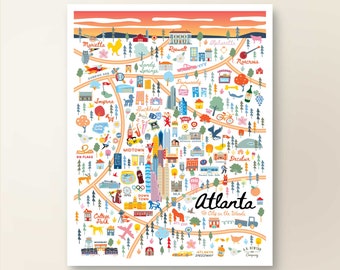This image displays a colorful, cartoony illustration that appears to be a playful and detailed map-like artwork of Atlanta. The artwork, set against a white background, showcases various vibrant elements in red, blue, yellow, orange, and green. At the bottom right corner, "Atlanta" is written in black cursive. The illustration features a whimsical collection of roads, cars, landmarks, skyscrapers, little trees, and buildings, each representing specific locations and features of Atlanta. Notable areas such as Marietta and Dunwoody are labeled, indicating key suburbs and sections of the city. At the top, a town hall is set against a red and orange sky with white clouds. Additionally, there is an airplane visible at the bottom left, likely representing the airport. This detailed and lively depiction captures the essence of Atlanta through a series of charming and imaginative drawings.